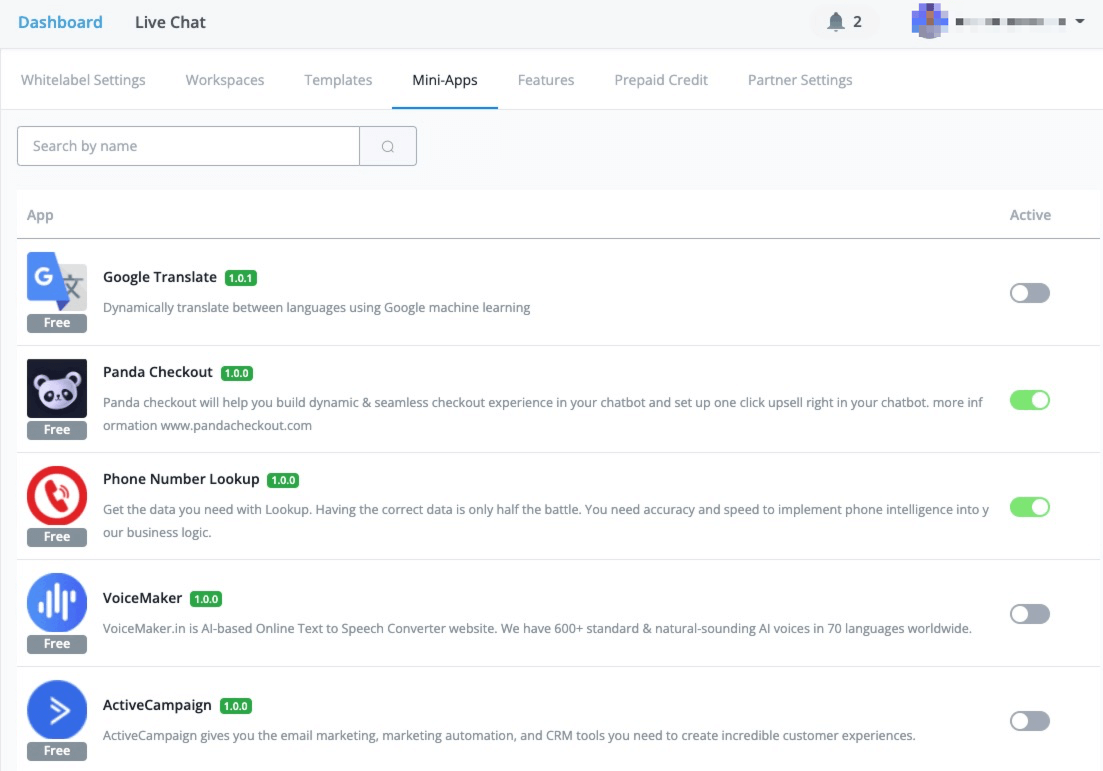This is a detailed screenshot of a computer screen displaying a software interface. At the top, there's a gray rectangular header containing the words "Dashboard" in blue print next to "Live Chat" in black print. Moving across the top bar, there's a bell icon with the text "2" beside it, likely indicating notifications.

Below the header, the screen is segmented into various sections. On the left, an entire column lists different applications. A centrally placed pixelated image showcases a sequence of black, white, and gray boxes followed by a section that incorporates blue and periwinkle colors. This area also features a drop-down menu.

Below this, a white horizontal bar spans the width of the screen, with the following options displayed in sequence: "White Label Settings," "Workspaces," "Templates," and "Mini Apps." The "Mini Apps" option is highlighted and underlined with blue. Additional categories include "Features," "Prepaid Credit," and "Partner Settings."

Towards the bottom, there is a search bar labeled "Search by name" with a clickable magnifying glass icon for searching. To the right, there is a section labeled "Active" where various toggle switches are displayed. These toggles are initially gray, indicating they are off. When switched on, the background of the toggle turns green, shifting the slider ball to the right.